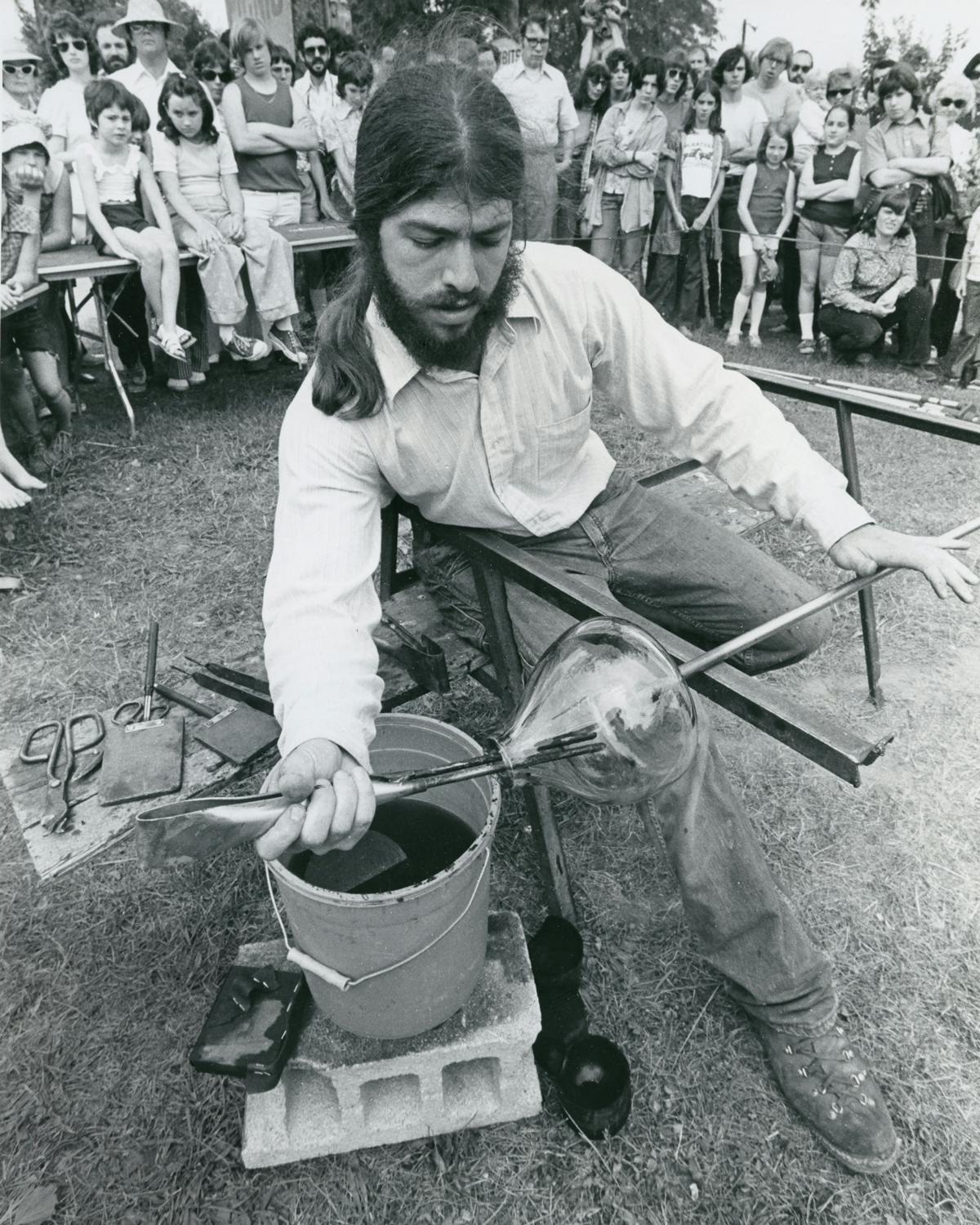This black-and-white photo, likely taken in the late 70s or early 80s, captures a man engaged in the intricate craft of glassblowing. The scene is vividly detailed with the man, a Caucasian with long hair tied back in a ponytail, a full beard, and mustache, as the focal point. He is seated on a metal-framed chair, intently working with molten glass. Dressed in a white button-down shirt and jeans with boots, he extends his right leg while his left leg is bent behind him.

In his hands, he holds a metal rod with molten glass forming a bulbous shape at the end, using the chair's arm to roll it. A bucket of water rests on a brick beside him, essential for the glassblowing process, along with numerous tools scattered on the ground. He meticulously manipulates the glass, rolling and shaping it with precision.

Behind him, a large crowd composed of men, women, and children watches intently. The onlookers, some seated on tabletops and others standing, are deeply engrossed in the demonstration. Many wear sunglasses, suggesting a bright day. The clothing styles and overall atmosphere hint at a vintage era, adding a nostalgic layer to this remarkable snapshot of a traditional art form.